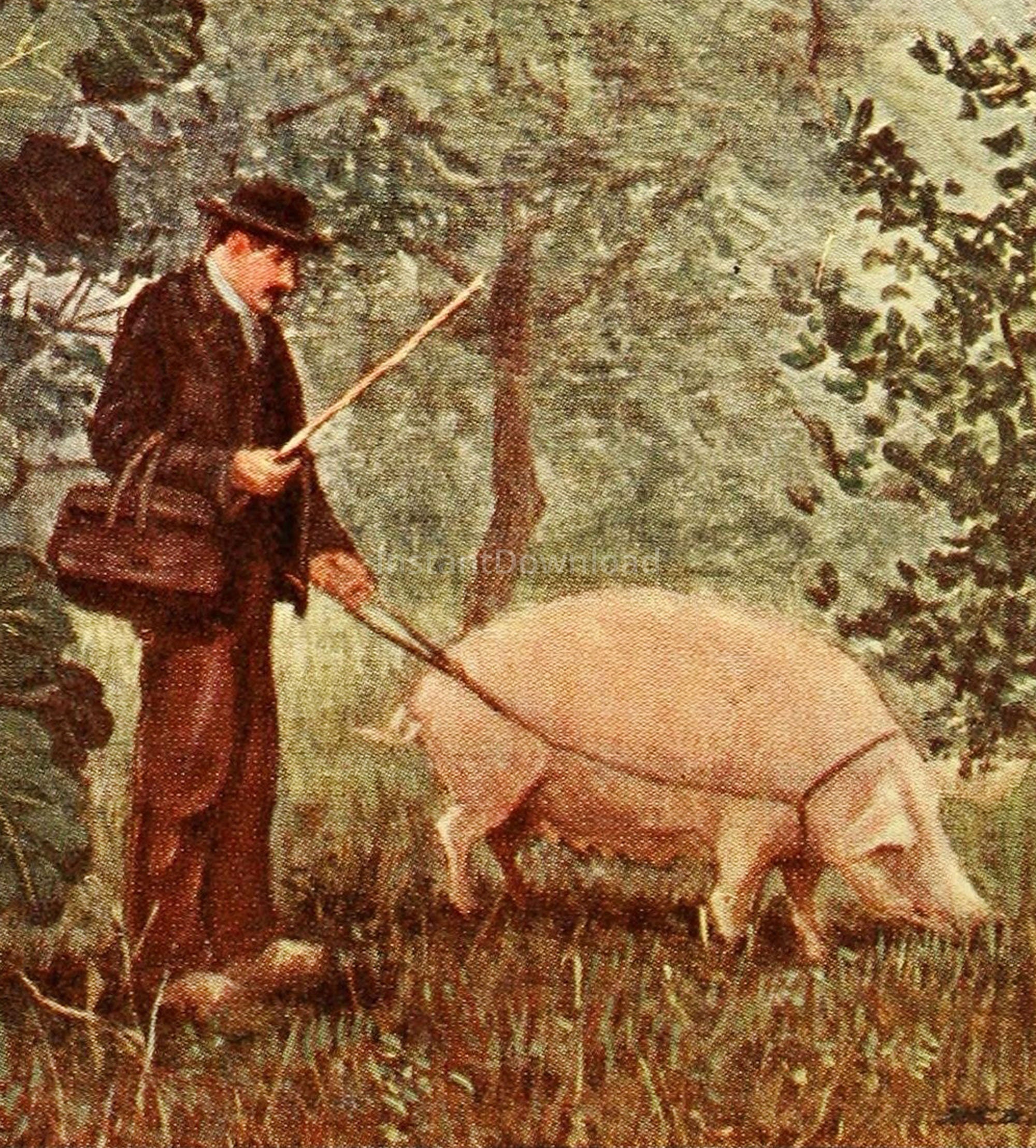This is an image of a painting depicting a man walking a pink pig on a leash. The man, who appears to be dressed in a dark coat that looks brown and reddish-brown pants, is wearing a black top hat. In his right hand, he holds a tan-colored cane, and around his left forearm, he carries a small brown bag or statue with straps. The pig, featuring a bunch of udders indicating it's a female, is on a leash held by the man's left hand. The scene is set in a forested area, with grass below them and trees and bushes painted in the background. There is a watermark on the image with some unreadable text.